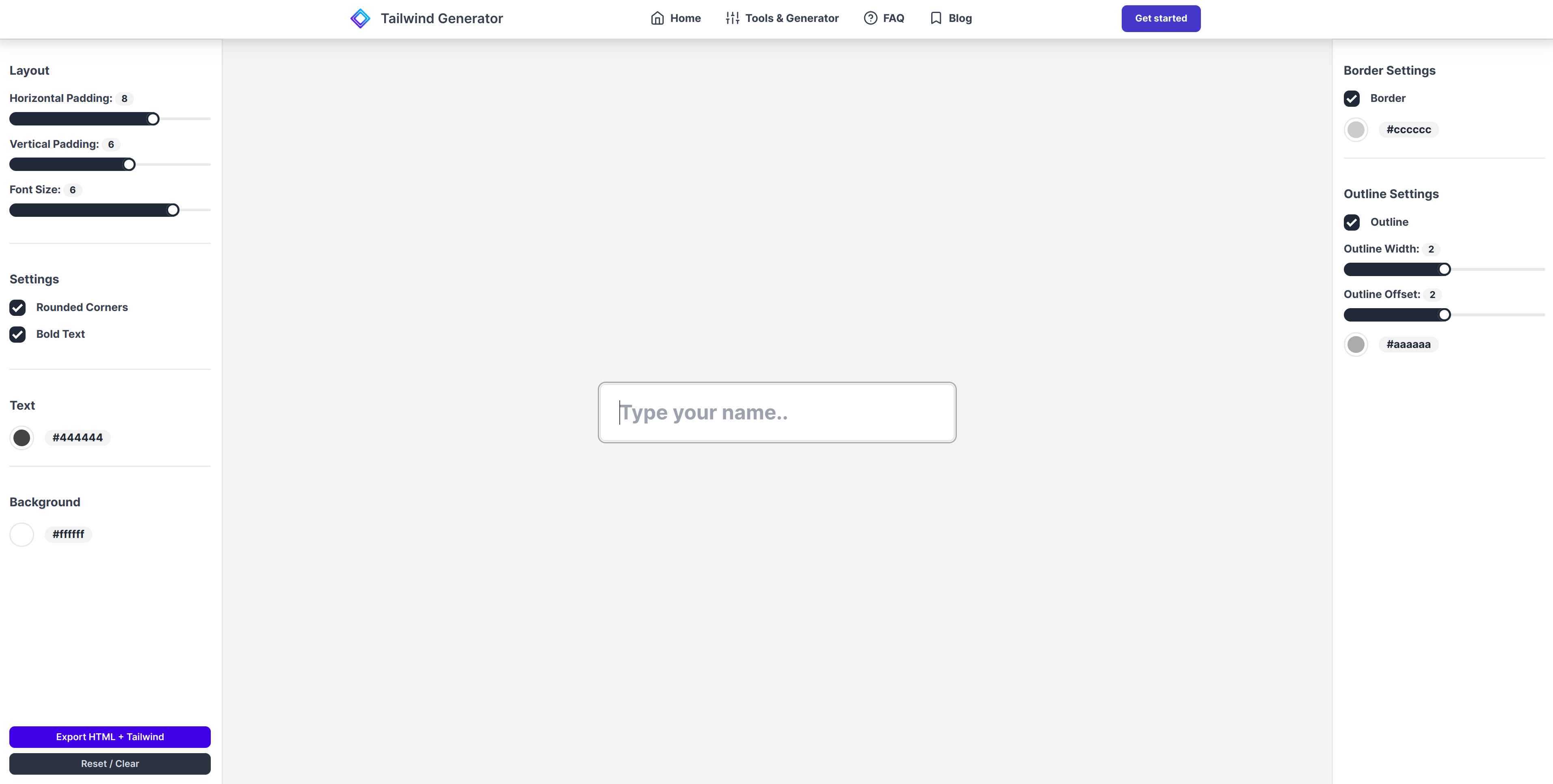This screenshot captures a detailed view of a web-based design tool interface named "Tail Wind Generator". Running along the top toolbar, the interface features navigation options including a "Home" button, "Tools", "Generator", "Help" section, "FAQ", and a "Blog" section, along with a prominent blue "Get Started" button. 

The main body of the webpage displayed is predominantly gray and includes a central text box prompting the user to "type your name". 

On the left-hand side of the screen, a secondary toolbar provides various customization options: 
- "Layout"
- "Horizontal Padding"
- "Vertical Padding"
- "Font Size"

Below these options, the "Settings" section lists checkboxes for "Rounded Corners" and "Bold Text", both of which are currently checked. Beneath "Settings", there are additional options labeled "Text" with a clickable circle, followed by "Background" with another clickable button, an "Export HTML" button in blue, and a "Reset Clear" button in black.

On the right side of the screen, there's a section titled "Border Settings". The "Border" option is checked, and below it, another checkbox without descriptive text is available. Further down, "Outline Settings" include several adjustable features:
- An "Outline" checkbox, which is selected
- "Outline Width" and "Outline Offset", both equipped with slider bars

Lastly, there's an additional, unspecified button available for checking.

This structured user interface provides extensive controls for tailoring web elements, making it a robust tool for designers.